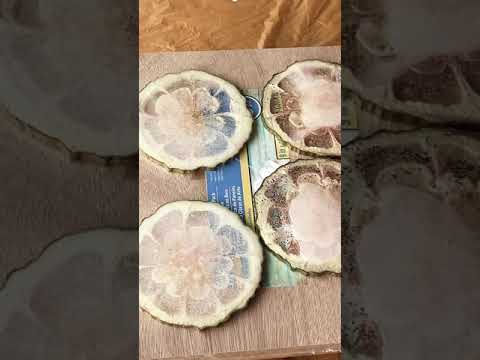The image displays four thin, semi-translucent slices of what appears to be dried fruit or plant matter, resembling citrus segments with a distinct flower shape in the center. The slices exhibit tones of white, beige, and clear, giving an impression of fragile, preserved natural elements. They are arranged on a small wooden board, which itself is placed on a beige, cloth-like background. The wooden board still has a blue, green, and gold label affixed to it. This ensemble is presented vertically within the image, flanked on the sides by enlarged, grayscale versions of the central image, creating a bordered effect. The overall setup suggests an aesthetic arrangement, possibly in a kitchen or a similarly rustic setting.